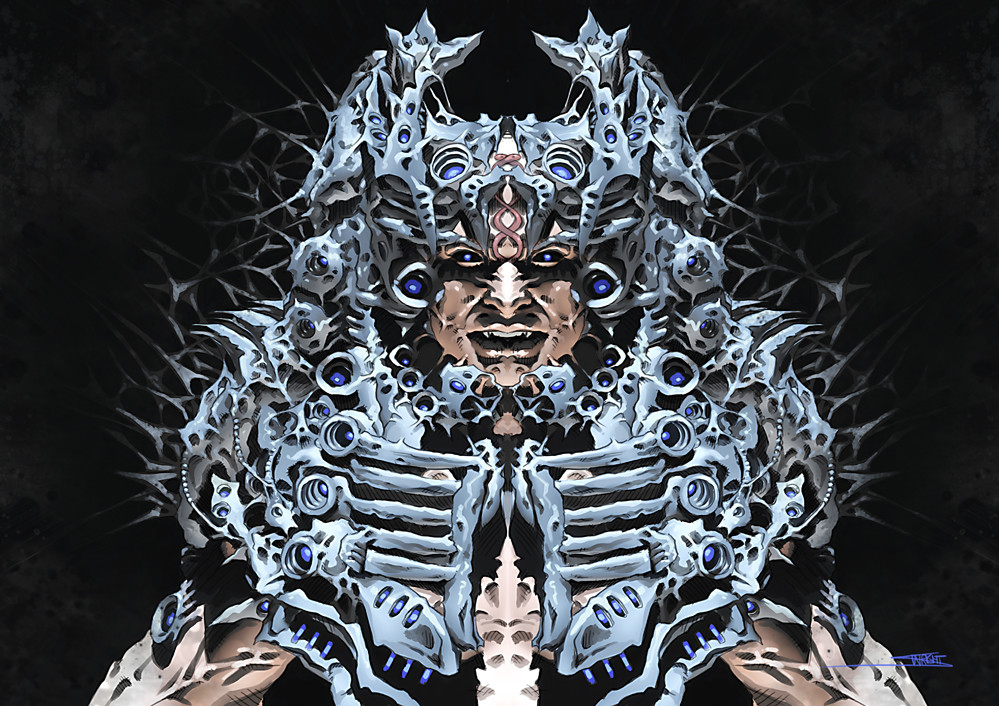This detailed, photorealistic drawing, signed by an illegible artist in the lower right corner, features a menacing figure set against a black background. The central focus is a diabolical-looking character with dark skin, fangs gleaming in a sinister grin, and deep blue eyes that emanate a piercing light. His face, marred with scars, is framed by an elaborate mask resembling bones, potentially fashioned from an ice blue, gray-toned material. This mask encases his head, extending over his shoulders and down to his chest, where an open ribcage with five bones on each side, connected by vertebrae-like elements, adds to the eerie and complex design. Brown, metallic plates, possibly shoulder pads, complement the mask, which is adorned with spiky, sharp, and barbed details. Each sharp edge reflects an almost steel-like blue tint, enhancing the dark and fanciful nature of this enigmatic image. The figure's form is further accentuated by small blue lights embedded within the armor, contributing to the overall sinister and graphic quality of the artwork.